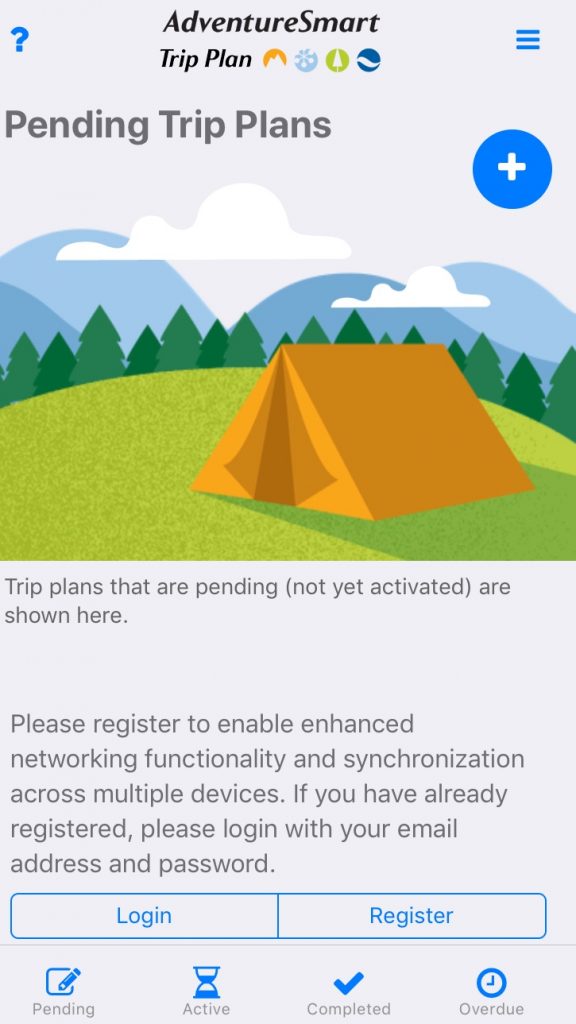Image Caption:

The image depicts a user interface related to camping and adventure planning. At the top, the phrase "AdventureSmart" is prominently displayed with the 'A' and 'S' capitalized. Below this, the italicized words "Trip Plan" are written. To the right, there are four icons symbolizing different elements of nature: mountains, snowflakes, a tree, and a wave. 

On the far left corner of the image, there is a blue question mark icon. In the top right corner, three horizontal blue lines are visible. Below the "Trip Plan" heading, on the left side, the words "Pending Trip Plans" are written. Diagonally to the right, there is a white plus sign inside a blue circle.

The central visual element is a cartoon illustration of an orange tent set on a hillside in a natural landscape. The scene includes two clouds in the sky, rolling blue hills, and several green trees.

Beneath the illustration, a message reads: "Trip plans that are pending (not yet activated) are shown here." Three lines down, another message states: "Please register to enable enhanced networking functionality and synchronization across multiple devices. If you have already registered, please log in with your email address and password." Below this, two blue buttons labeled "Log In" and "Register" are side by side.

At the bottom of the image, there are four categories: "Pending," "Active," "Completed," and "Overdue." Each category is represented by an icon: a sketchbook and pencil for "Pending," an hourglass for "Active," a check mark for "Completed," and a clock for "Overdue."